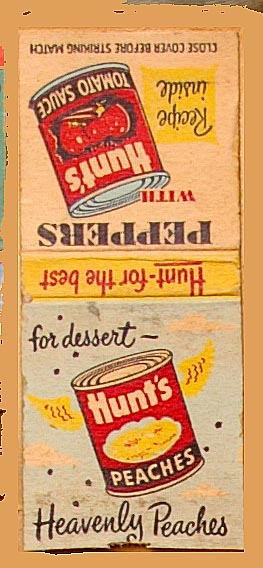The advertisement features a charming, vintage design with a light orange background. It is divided into two horizontal sections. The upper section contains an inverted rectangle with a yellow banner stating, "Hunt's - for the best," in red letters. Above this, the black, upside-down text reads, "peppers with," accompanied by an illustration of an upside-down can of Hunt's Tomato Sauce. The can's prominent red label contrasts with its silver top and edges, and a small orange square beside it declares, "recipe inside." 

The lower section showcases a delightful promotion for Hunt's Peaches. Nestled against a light blue corner, the cursive black text announces, "for dessert," alongside an angled can of Hunt's Peaches, which sits on an elegant white plate filled with juicy, yellow peaches. Beneath this display, another black script firmly asserts, "heavenly peaches." The ad's aged aesthetic is enhanced by its overall tan hue, emphasizing the nostalgic appeal of these classic Hunt's products.